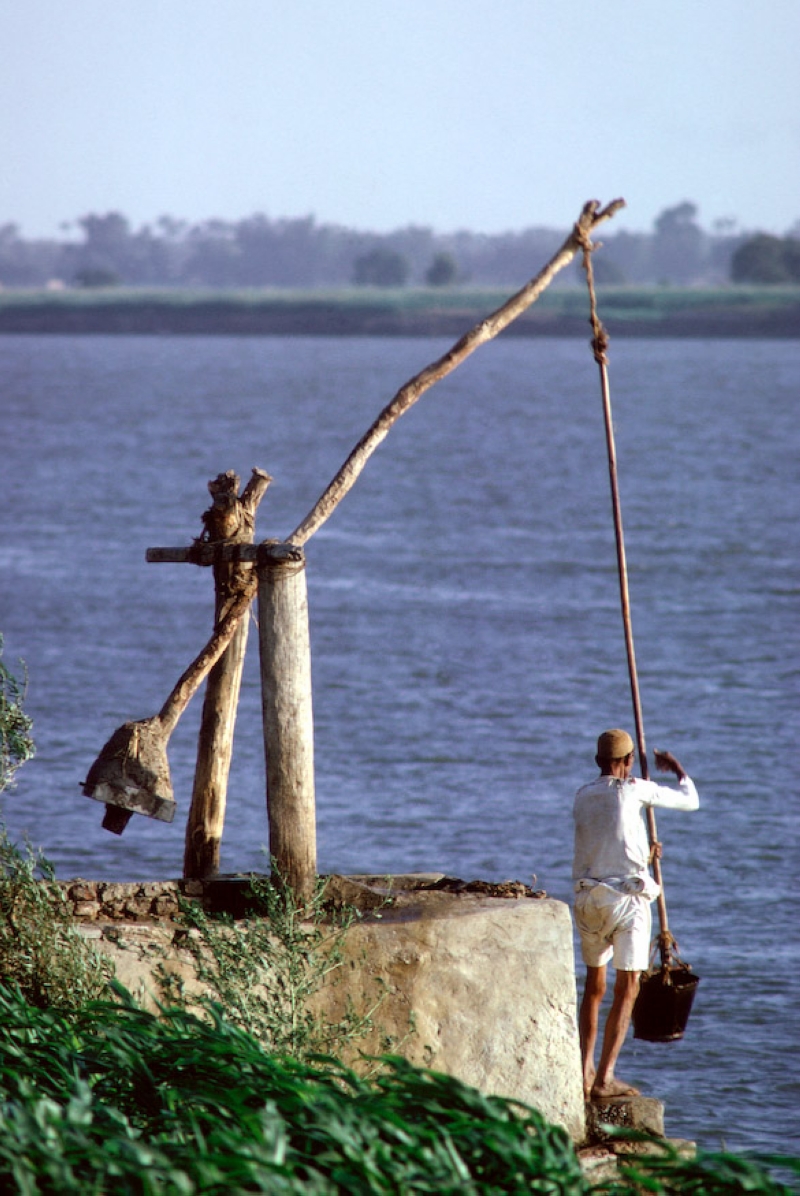In this photograph taken in a natural setting, a man dressed in a white long-sleeve shirt and white shorts is seen standing next to a wide body of water, which might be a river, lake, or even a sea or ocean scape. The water stretches out into the distance where a grassy ridge meets a forest line under a cloudy sky. In the foreground, dark green grass and leafy foliage frame the scene. Prominently featured is a roughly three-foot-tall stone structure with two wooden posts supporting a horizontal beam. Attached to the beam is a long wooden stick that swings like a pendulum. A rope hanging from the end of the stick holds a bucket, which the man is either lowering into the water or retrieving from it. This homemade contraption, possibly for collecting water or fishing, highlights the man’s interaction with the tranquil landscape.